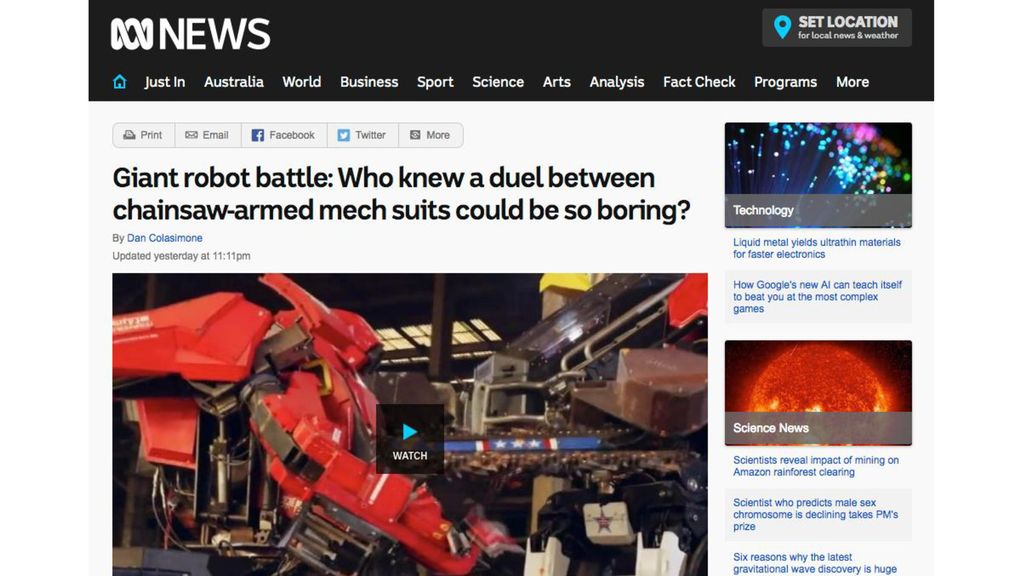The image displays a news interface with a black banner at the top. On the upper left corner, there is a white icon followed by the word "news." On the right side of the banner, there is a message reading "Set location for local news and weather" accompanied by a turquoise pin icon. Below the banner, a black background showcases several categories in white font: "Just In," "Australia," "World," "Business," "Sport," "Science," "Arts," "Analysis," "Fact Checks," "Program," and "More." To the left of "Just In," there is a turquoise house icon.

Under these categories, there are grey buttons with black fonts for "Print," "Email," "Facebook," "Twitter," and "More." 

The main headline reads: "Giant Robot Battle: Who knew a duel between chainsaw-armed mecha suits would be so boring?"

On the right side, there are several news snippets under different headings:
- **Technology**: "Liquid metal yields uranium materials for faster electronics."
- **Technology**: "How Google's new AI can teach itself to beat you at most complex games."
- **Social Science**: "Scientists reveal impact of mining on Amazon rainforest clearing."
- **Science**: "Scientist who predicts male sex chromosome is declining takes PM's prize."
- **Science**: "Six reasons why the latest gravitational wave discovery is huge."